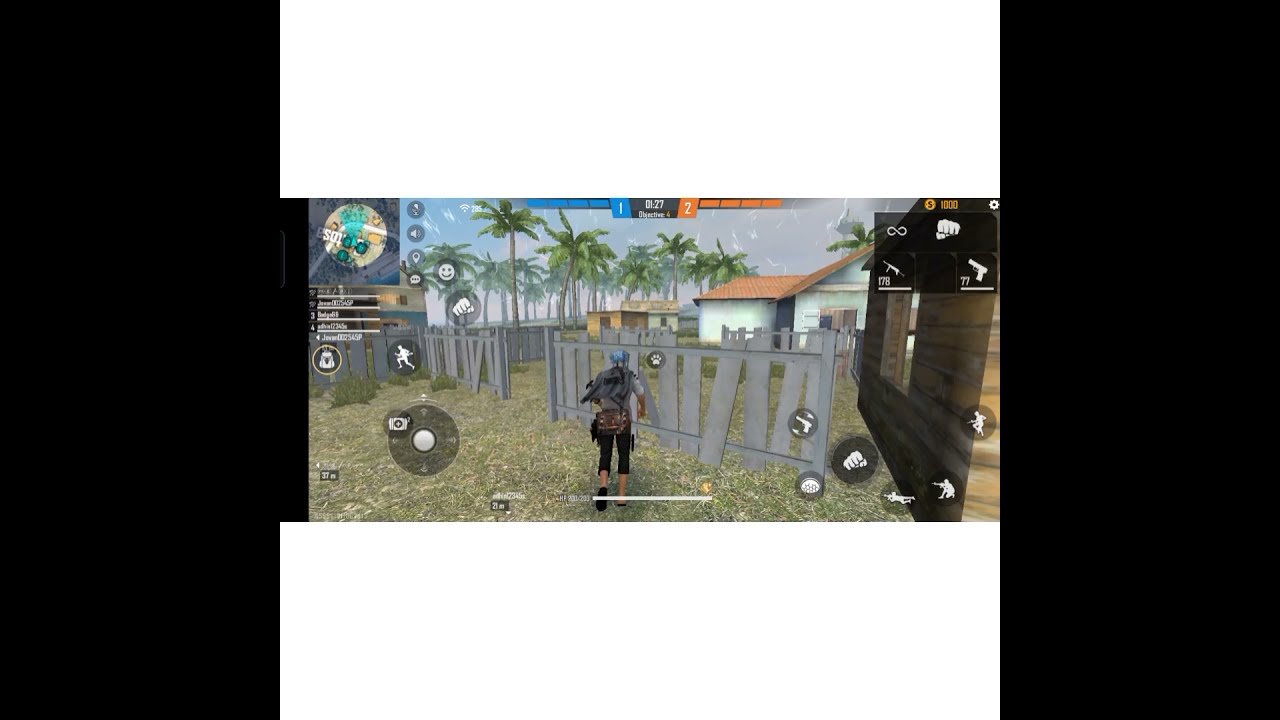The image is a detailed screenshot from a computer video game, prominently framed by horizontal white bars and vertical black bars. The central focus of the scene captures a man facing a broken gray wooden fence, dressed in black pants, a gray shirt, a blue hat, and carrying a gray backpack. Surrounding the character is a verdant landscape with grass and distant palm trees. In the background, there are two buildings: one is green with a single window, and the other nearer to the palm trees is light blue with red clay tiles and two windows.

The game interface is replete with interactive menus and icons. On the upper left-hand corner of the screen, there's a mini-map, while the lower left holds an analog stick for character movement. The right-hand side is populated with action buttons, including icons for a fist to punch, a gun to shoot, and additional options such as a hand and two more weapons. At the bottom, there’s a round circle icon with a camera, adding to the gaming controls. The detailed environmental setting and numerous in-game controls underscore the immersive experience of the game.